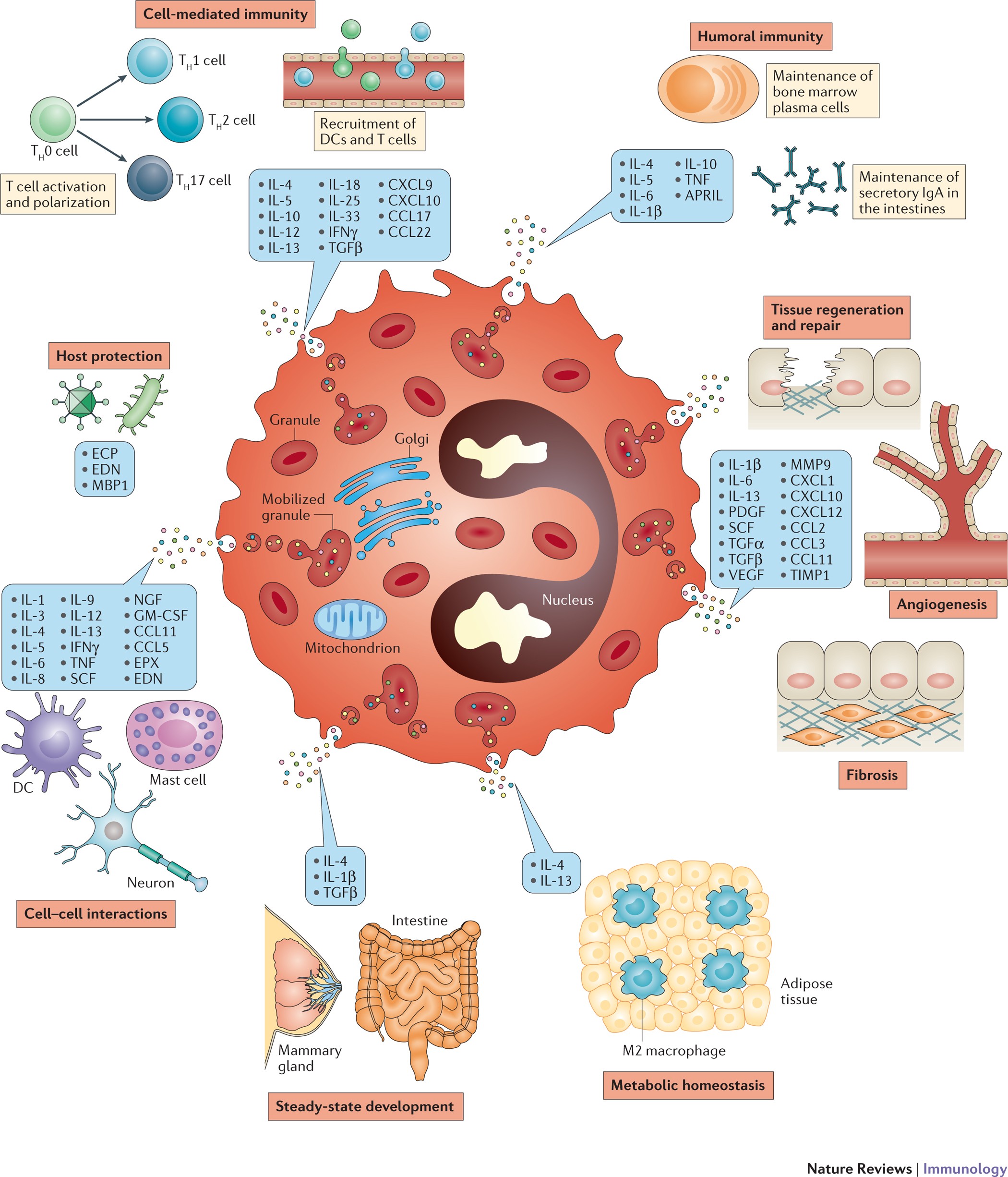This detailed diagram illustrates the complex interactions and functions within cell-mediated and humoral immunity. Central to the image, a stylized cell is depicted against a white background, detailed with various intracellular components: a jagged cell wall, red granules with darker centers, mobilized granules speckled with blue, white, and yellow dots, blue Golgi apparatus, blue mitochondria, and a uniquely shaped nucleus resembling a stylized telephone. Surrounding the cell are multiple color-coded word bubbles with annotations in blue text, denoting processes and interactions including "tissue regeneration and repair," "host protection," "cell-cell interaction," "steady state development," and "metabolic homeostasis."

The image also features various anatomical and physiological elements such as an artery, mammary gland, intestine, adipose tissue, angiogenesis, and fibrosis, highlighting interconnected biological systems. Abbreviations and terms like mass cells, DC (dendritic cells), and neurons are annotated to emphasize the diverse interaction between cellular and systemic processes. Overall, the diagram provides a comprehensive visual representation of the immune system’s multifaceted mechanisms, underscoring the intricate cellular activities and their broader implications for organismal health.